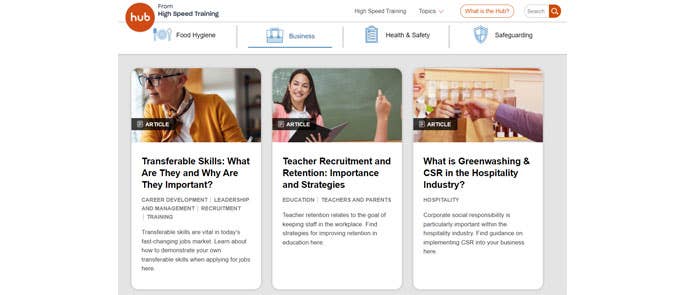### Comprehensive Caption:

The image is a screenshot of a web page from "High Speed Training," identified by an orange circular badge with "HUB" written in white letters on the left side. Next to this badge is the site’s name, "High Speed Training," followed by a navigation menu with a "Topics" drop-down arrow and a white button labeled "What is the HUB?". To the right, there's another white button featuring an orange section at the corner, which reads "Search".

Beneath this navigation bar, a blue icon featuring a fork, plate, and spoon is labeled "Food Hygiene". Next to it, a briefcase icon represents the "Business" section, and an icon of a notebook pertains to "Health and Beauty". Following these icons is another section labeled "Safeguarding".

The main content below these sections is divided into three windows:

1. The first window displays a woman with short blonde hair wearing black glasses, an orange jacket, and a white shirt. It is captioned "Transferable Skills: What They Are and Why They Are Important".
   
2. The second window features a woman with long black hair in a pink jacket and white shirt, holding a notebook.

3. The third window shows a woman carrying grocery bags next to a headline that reads "Why Greenwashing and CSR Matter in the Hospitality Industry".

This descriptive caption provides a detailed overview of the web page's structure and content.